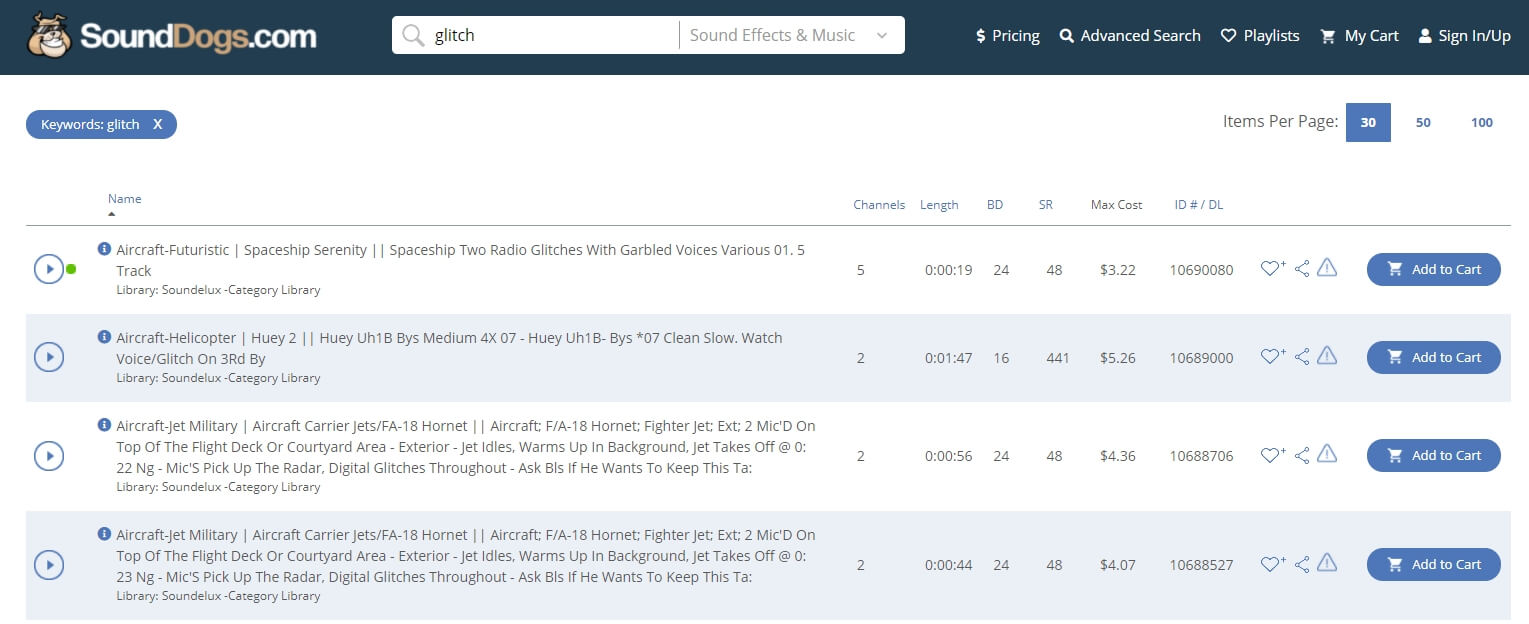The image showcases a webpage from SoundDogs.com, a site specializing in sound effects and music. At the top, the website's name "SoundDogs.com" is prominently displayed. Below, a search box contains the terms "Glitch, Sound Effects and Music." The navigation bar includes various tabs such as "Pricing," "Advanced Search," "Playlists" (accompanied by a heart icon), "My Cart" (indicated by a cart icon), and "Sign In/Up" (with a person's head outline).

Further down, there's a section labeled "Keywords: Glitch" with options to select the number of items per page (30, 50, or 100). The content area lists different sound effects, including "Aircraft Futuristic," "Spaceship Serenity," "Spaceship 2 Radio Glitches with Garbled Voices," "Various 0.15," and "Track." Each listed item has a blue play button and detailed attributes, such as:

- Channels: 5
- Length: 19 seconds
- Bit Depth (bd): 24
- Sample Rate (sr): 48
- Max Cost: $3.22
- ID: 10690080

Additional icons for each item include a heart icon for saving, a share button, and a triangle with an exclamation mark. A blue "Add to Cart" button is also available. The overall page features a white background with black text.